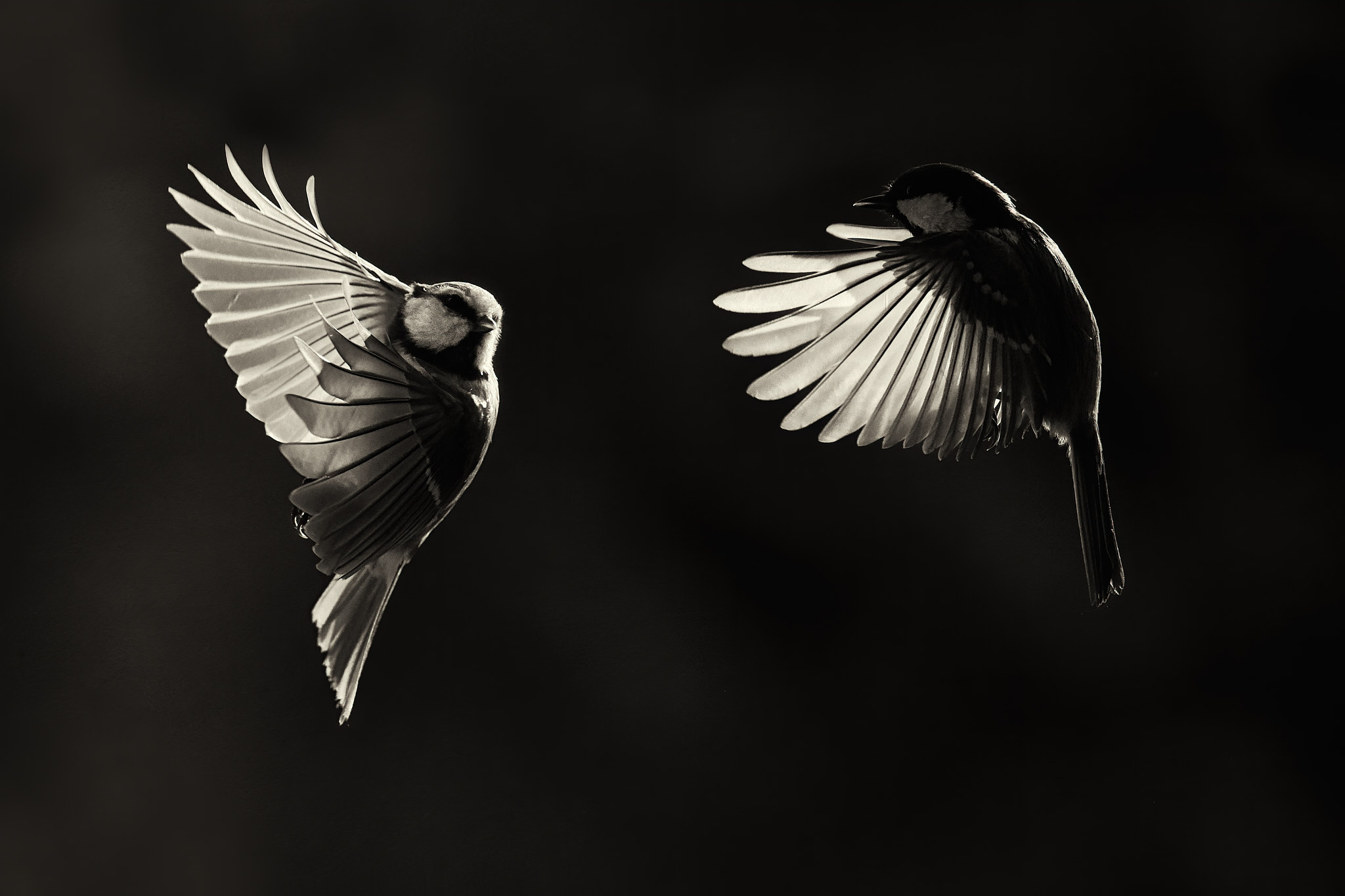In a striking black and white photograph, two birds are captured mid-flight against a completely black background. The bird on the right, illuminated by a bright light from the top right corner, faces towards the left. Its translucent wings, lit from behind, reveal an ethereal glow. Simultaneously, the bird on the left appears to be twirling to its right to meet the other bird. Caught mid-turn, it extends its left wing while its right wing crosses over its body, hinting at dynamic motion. Both birds’ wings are partially closed as they move, creating a harmonious rhythm in their flight. The absence of any text allows the focus to remain solely on the elegant dance of the birds, with shades of white, gray, and black adding depth to the monochromatic scene.